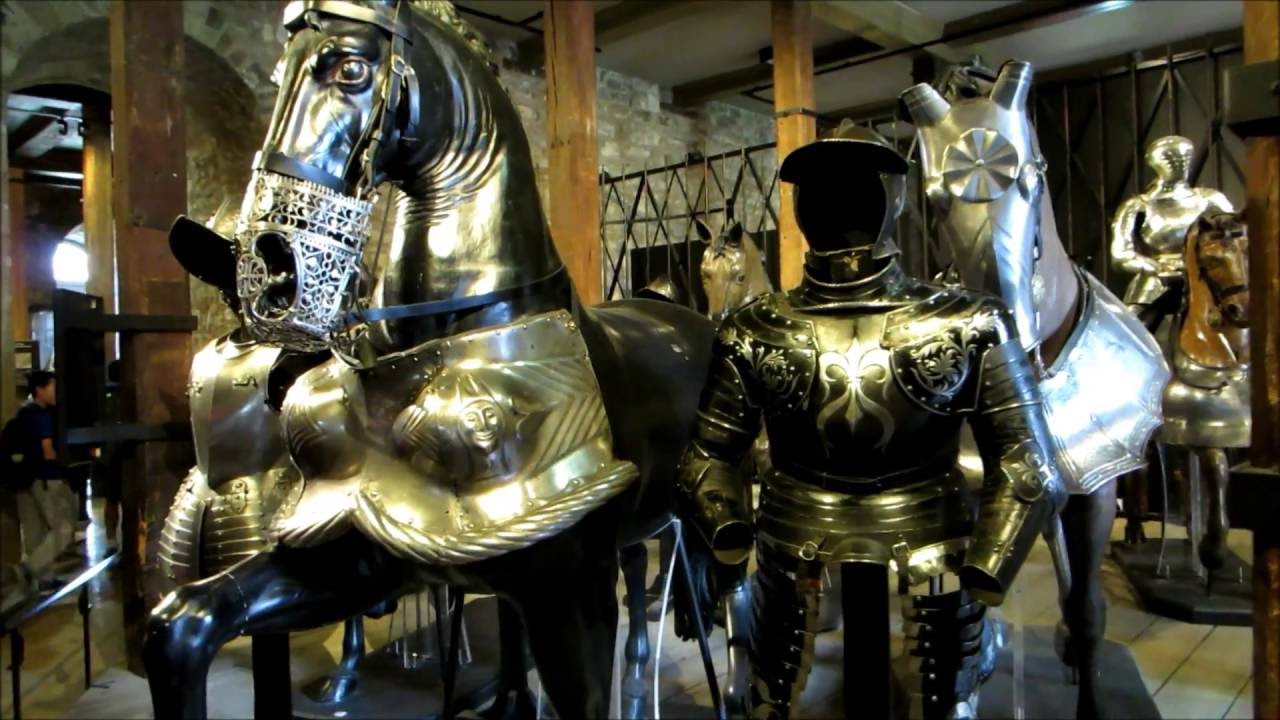The photograph, taken inside a museum, showcases an impressive array of armor exhibits from various historical periods, evident by their diverse designs. The room features white squared tiles with black routing on the floor and is sectioned by black expandable fencing. The walls are constructed of squared gray stone, emulating the interior of a castle, with a prominent stone archway on the top left hinting at an adjoining room. Numerous sturdy brown wooden pillars support the ceiling.

On display are four horses adorned with intricately designed armor. The closest horse sports a metal filigree bridle and muzzle piece, reminiscent of a feed bag. This horse, along with adjacent human armors, is predominantly covered in gold-plated armor. Another horse on the right showcases silver armor, and further right, a fully armored rider sits astride another armored horse, exuding a sense of readiness for battle. The far right edge of the photograph catches a glimpse of a fourth horse’s head adorned with armor. Both gold and black elements feature prominently in the armors, adding to the overall regality and historical significance of the displays. Additionally, a visitor can be seen exploring the exhibit, adding a touch of contemporary context to this historical showcase.